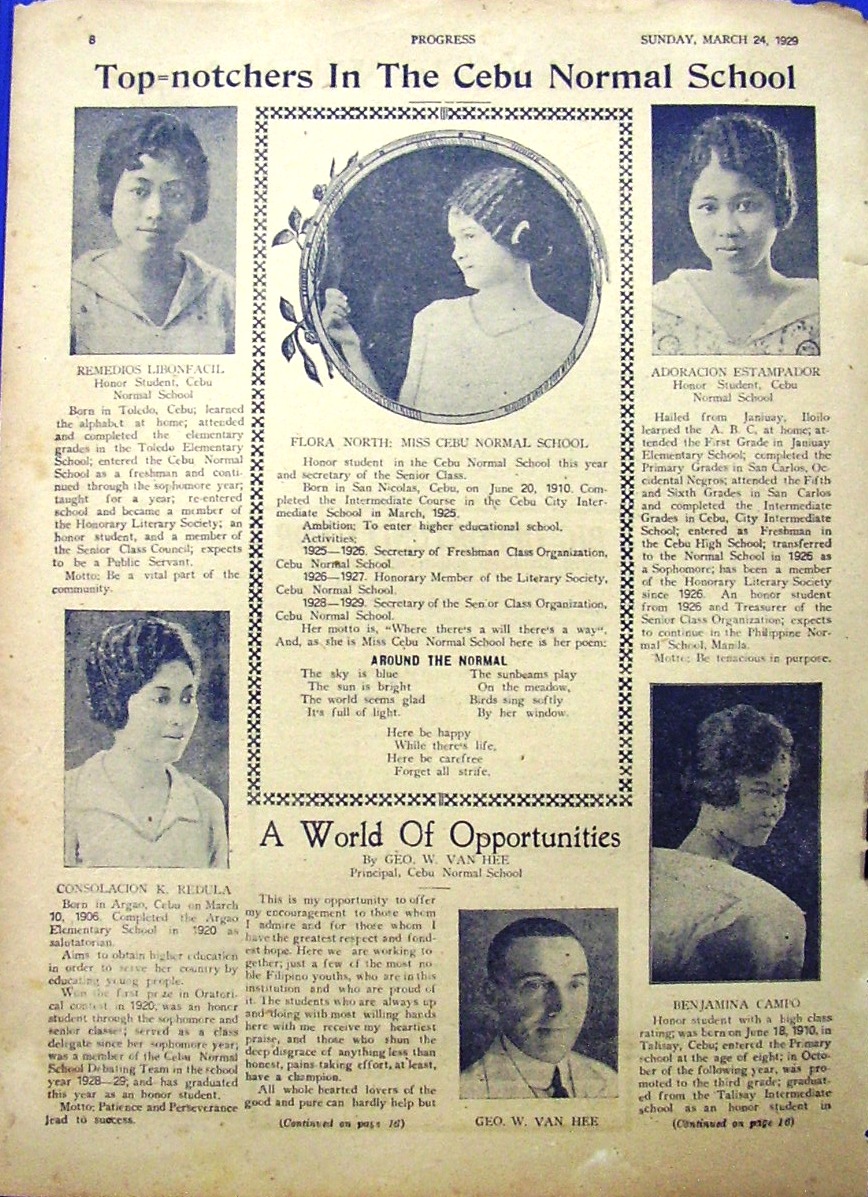The image is a scan of an old, yellowed piece of paper from a publication dated Sunday, March 24th, 1929, possibly from a yearbook or an old magazine. The page is headlined with "Top Notchers in the Cebu Normal School" in large black letters. The page number "8" is visible at the top left, while "Progress" is at the very top, indicating the publication's name.

There are multiple black-and-white photographs of people arranged on the page, mostly women, with descriptive articles or bios beneath each photo. The top left corner features a photograph of a woman, identified as Remedios Libin Fasil, an honor student from Cebu Normal School, with brief biographical details such as her birthplace in Toledo, Cebu, and her early education at home.

In the top center, there's a round photograph of Flora North, labeled "Miss Cebu Normal School." At the bottom center of the page, there is a photograph of a man, G.O.W. Vaughn He, accompanied by a snippet of information concerning his connection to the school. The images and accompanying text appear to share brief biographies and accolades of the featured individuals, all of whom are associated with Cebu Normal School.